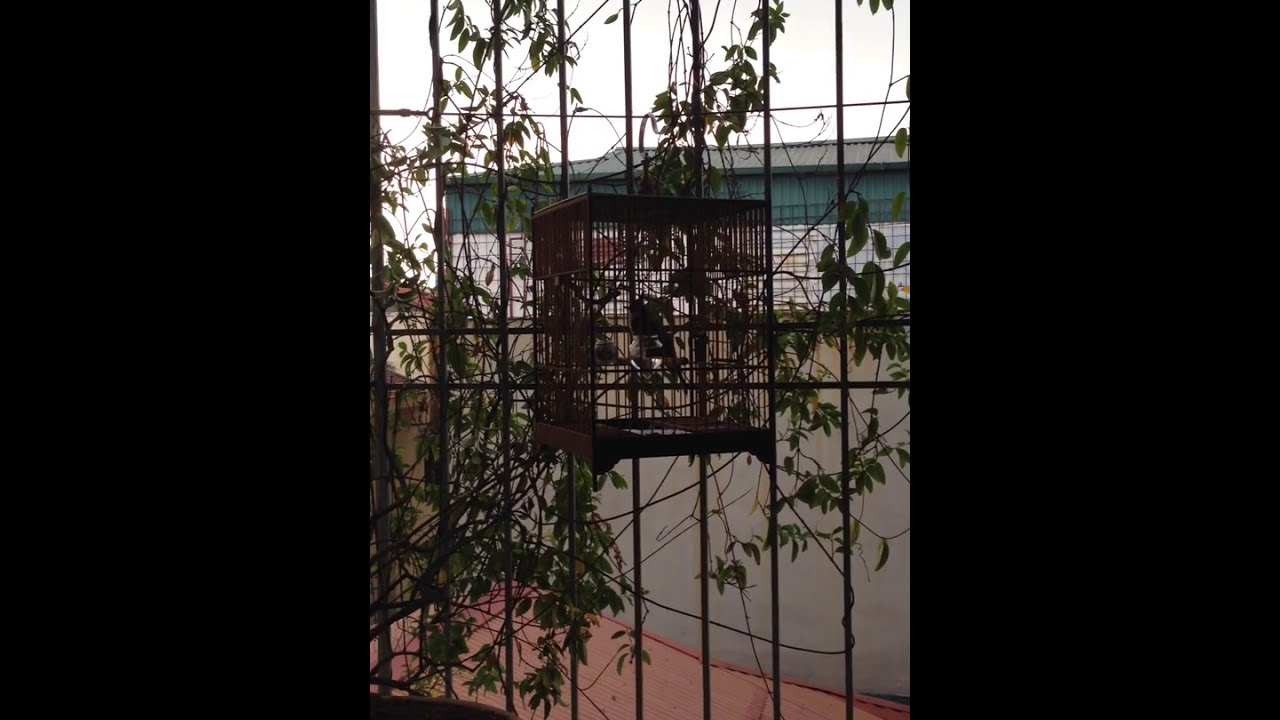The photograph showcases an outdoor recreational area dominated by a prominently centered black birdcage suspending from an unseen overhead structure. The birdcage, with its vertical and horizontal black bars, houses at least two or three birds. Directly behind the birdcage is a black wire fence characterized by thin, long vertical wiring and supported by horizontal bars. This fence is partially obscured by a green vine that entwines itself around the black wiring. Beyond the fence, a red-bricked curved walkway appears at the lower edge, leading to a green paved patio area. Farther in the background, a gazebo or tented structure with a peaked, blue roof and open sides stands under a gray, overcast sky. There is additional black framing along the left and right edges of the photograph, narrowing the view and emphasizing the central elements. The scene is lush with surrounding trees and foliage, adding a vibrant mix of greenery that intertwines with the structured elements of the birdcage and fencing.